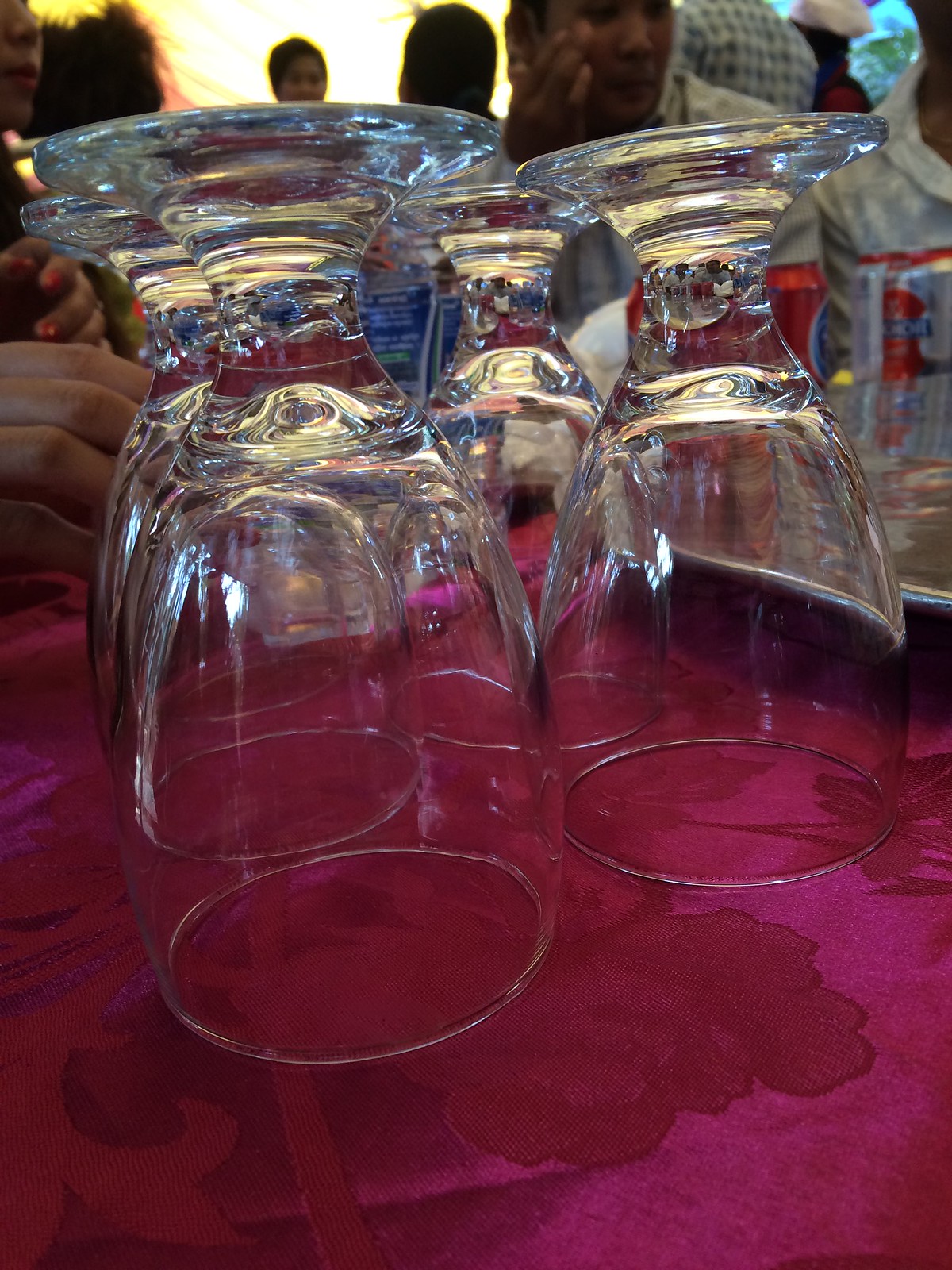This indoor colour photograph captures a detailed and vibrant scene, likely inside a restaurant. The image prominently features four upside-down water glasses, each with a thick and sturdy base, wide and slightly ballooned cups, and short, wide stems. These glasses are arranged in two rows of two on a shiny, satiny maroon tablecloth adorned with an embossed floral pattern. Small pools of water are visible underneath them, suggesting they were recently washed and set out to dry. To the left of the glasses, a hand with visible fingers can be seen, and to the right, a silver tray with a red can and an aqua-colored bottle stopper is partially visible. The background blurs slightly, revealing the heads and silhouettes of several people who appear to be sitting at tables, engrossed in their own activities. One person is distinctly seen with their hand raised near their face, donned in orange nail polish, and another is glimpsed wearing a blue and white shirt. The upper left corner of the image is illuminated by a soft yellow light, enhancing the overall warmth of the indoor setting.